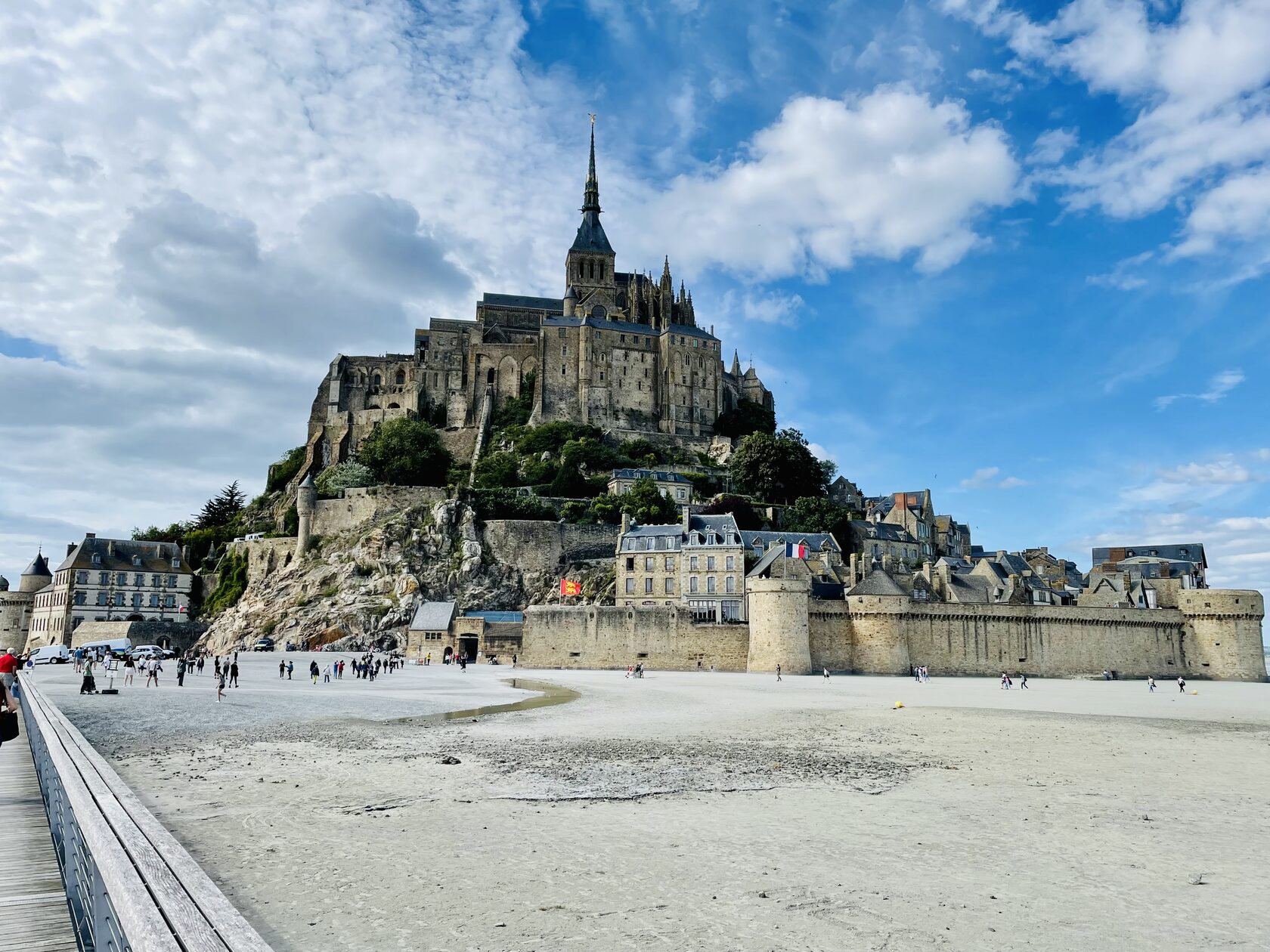This outdoor daytime photograph vividly captures a medieval stone castle with slate pitched roofs, perched atop a rocky, six- to seven-story mound. The castle, characterized by its weathered tan to brown color and a lofty central spire rising into a blue sky adorned with cotton candy-like clouds, evokes a sense of historical grandeur. A flag, possibly French, flutters in the breeze, adding to the charm of the scene. 

In the foreground, an expanse of sand suggests that the photo might have been taken from a pier, looking back toward the shore. A prominent stone seawall with rounded corners separates the sandy beach from a small village nestled at the foot of the hill. To the left, a white building marks the edge of the village, where several people are seen walking around on the sand. The village includes several stone buildings and houses, with the formidable castle towering above, dominating the landscape. The combination of medieval architecture, scenic natural elements, and bustling village life creates a picturesque and detailed portrayal of this remarkable location.